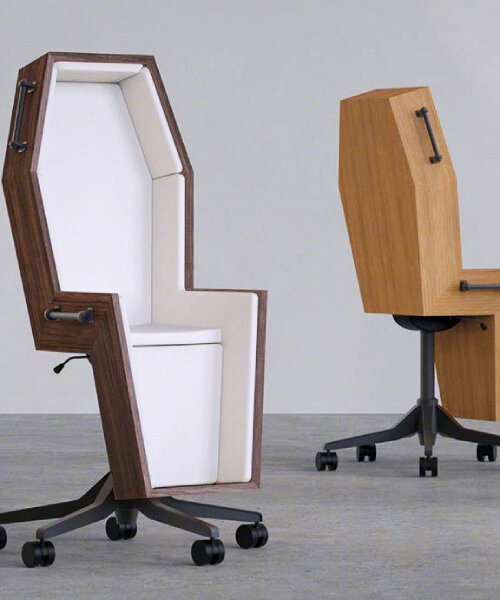This color photograph features two uniquely designed office chairs that mimic the appearance of upright coffins. Each chair is equipped with five rolling wheels, making them functional for an office setting. The backrests and bases of the chairs both follow a coffin's shape, with an angled section at the base to accommodate seating. 

The chair on the left is crafted from darker stained wood and showcases a white interior. Two black handles are prominently affixed—one near the top where your head would rest, and one in the middle of the back support, consistent with traditional coffin handles. 

The chair on the right features a blonde-colored wood and is turned away from the viewer, obscuring its interior. Like its counterpart, it also has handles: one at the upper middle and another at the lower middle, resembling those you'd find on a real coffin. 

Both chairs are situated on what appears to be a concrete floor, with no visible writing or people in the image, making it suitable for a brochure or magazine layout. The juxtaposition of the office functionality and the coffin design creates a striking and unusual visual effect.